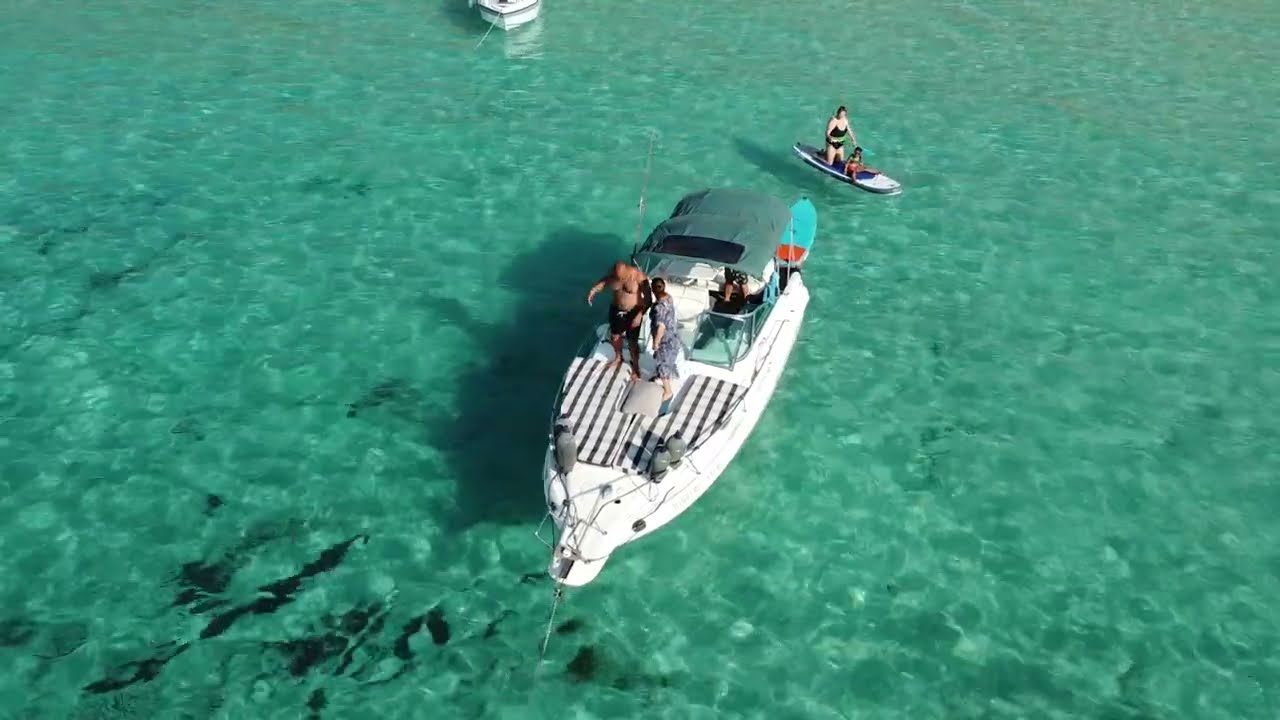An aerial view captures a vast water body with a vivid turquoise hue, filling the entire frame and revealing subtle ripples hinting at a mildly windy day. Dominating the center of the image, a white boat with a green roof is prominently featured. Two individuals stand on the deck, while a third person, possibly the boat's operator, is partially visible behind the deck's window. Adjacent to this boat, slightly to the top left, is a smaller paddleboard carrying a woman and a child, the latter wearing a distinctive red life preserver. The paddleboard, adorned in blue and white, contrasts against the green-black swimsuits of its passengers. Further into the background, barely within the frame, the bow of another boat is just visible, potentially anchored, suggesting more aquatic activity beyond the immediate scene.